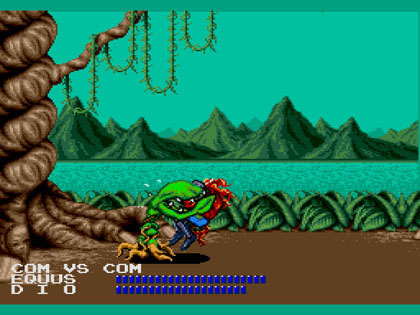This image depicts a 2D, pixelated graphic from an old DOS computer video game set in an outdoor environment. The background showcases a teal blue sky above green mountain peaks, which are reflected in a body of water a shade darker than the sky. The foreground features brown ground terrain sprinkled with leafy plants and a prominent twisted brown tree with elongated roots. A green vine dangles over a single tree branch. Central to the image is a troll-like creature resembling a Venus flytrap, with a big green head and pronounced white teeth, devouring a character with long red hair, whose boots stick out from the plant. The bottom left corner of the image displays white text reading "COM vs COM" and "Equus Diomedes," accompanied by blue life bars, indicating the health status of the characters.